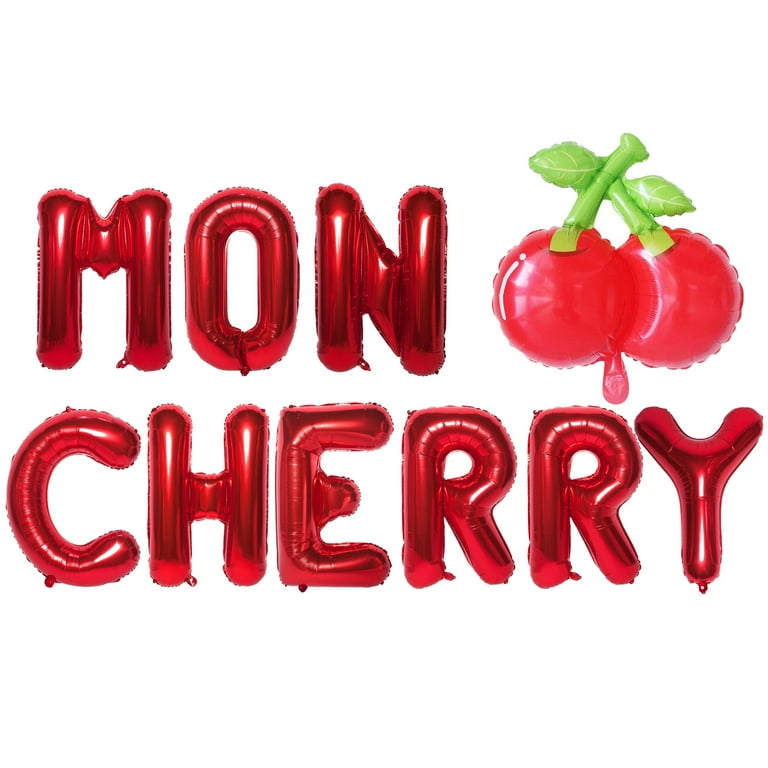The image is a detailed digital illustration in landscape orientation, featuring the words "Mon Cherry" rendered in large, inflated red balloon-like letters with reflective surfaces. The text is aligned to the left, with "Mon" positioned above "Cherry." To the right of the word "Mon," there is a vibrant depiction of two glossy cherries with scalloped edges, their green stems crossing with individual green leaves at the top. Red drops suggestive of dripping cherry juice or moisture are visible below the cherries and at the bottom of each letter, enhancing the visual appeal. The illustration has a 3D effect, making the letters and cherries appear three-dimensional and puffy. The entire composition, set against a white background, gives a striking and mouthwatering appearance, reminiscent of shiny mylar balloons filled with helium.